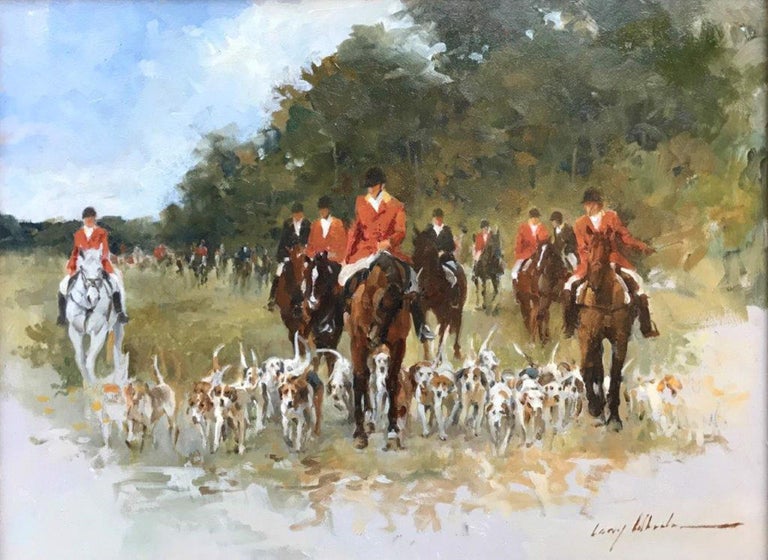The image depicts an intricate watercolor painting on a rectangular canvas, signed in the bottom right corner. The scene captures a bustling group of equestrians, elegantly attired in traditional fox hunting outfits. The riders don black or brown coats paired with white shirts and trousers, complemented by knee-length black boots and black hats. Mounted on horses of varied colors — predominantly brown, with some white and a few black horses in the background — they are accompanied by around 20 to 30 beagles, predominantly gathered in the center of the image. The background reveals an expanse of trees to the right and a clear blue sky, enhancing the sense of a crisp, early morning hunt amidst a picturesque landscape.